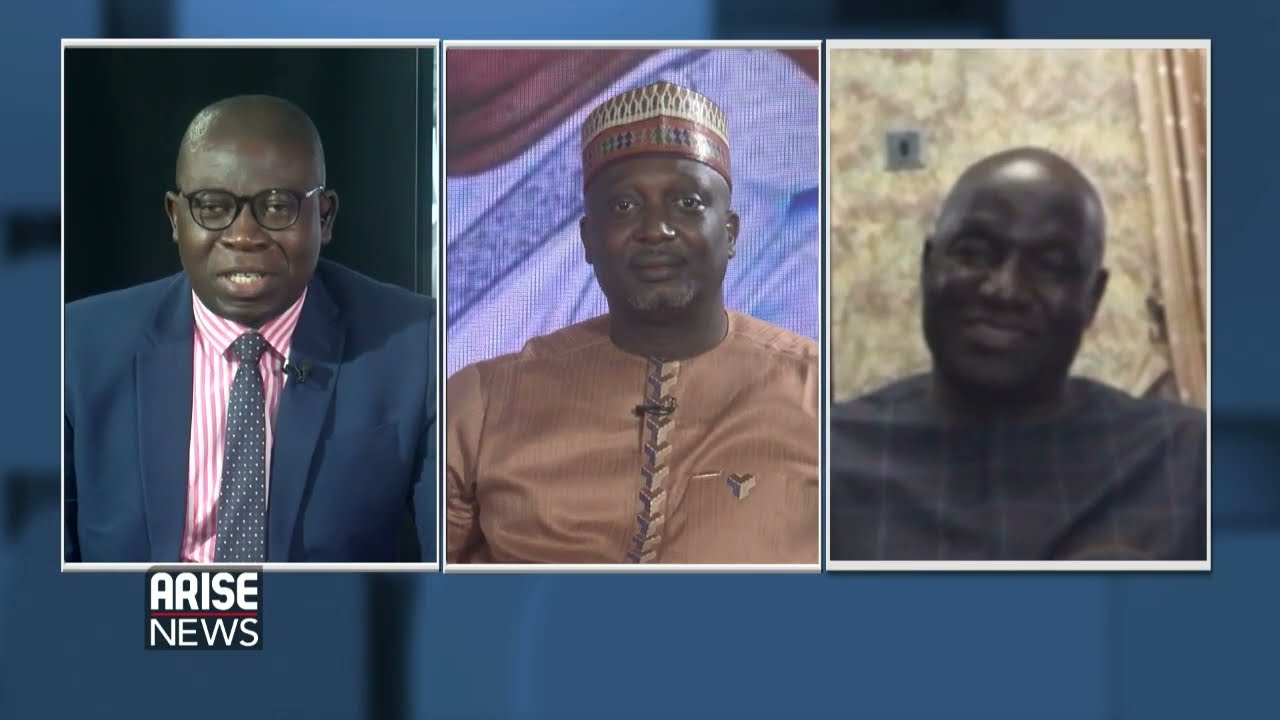The image is a screenshot of a TV news program, showcased on a news website with a dark blue background. In the lower-left corner, the text "Arise News" appears in white font with a red stripe between the words. The image features three Black men in separate frames, suggesting they are being interviewed remotely.

The man on the left is dressed in a dark blue suit, paired with a pink and white striped shirt and a tie with dots. He is bald, wears black circular glasses, and appears to be speaking, as his mouth is slightly open. The background behind him is black.

The central figure is adorned in a golden-brown outfit with a lace-up front, and he wears a distinctive multi-toned hat that resembles a turban with a possible snakeskin pattern on the top and a red and black design at the bottom. His background features wavy blue and white fabric with red linen material above it. He also appears to be wearing a microphone.

The man on the right is wearing a long black shirt. Although his image is slightly blurry, he is bald and seems to have a blurred background with a gold-colored curtain or wall. He is smiling and his photo is cropped at the shoulders.

The overall alignment and setting suggest a formal news interview or discussion with a clear, visually structured layout.